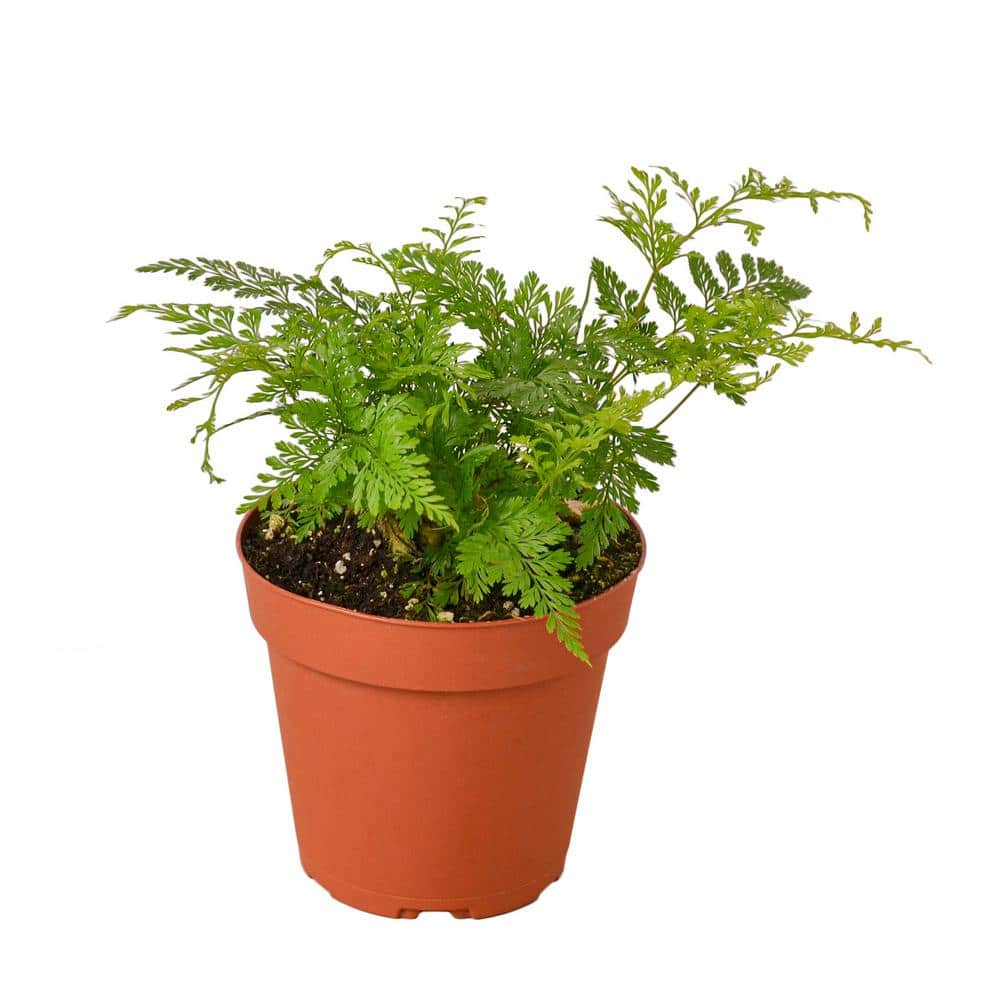This photograph showcases a healthy and vibrant green fern-like plant potted in a rich orange, round planter. The planter has a slightly wider rim at the top and is filled with dark brown soil interspersed with white specks. A few dried leaves are also visible on the soil. The delicate fern sprigs, boasting numerous little leaves, lend a light to medium green hue to the scene. The image, set against a plain white background, is captured from a slightly downward angle, emphasizing the plant's lush and graceful foliage.